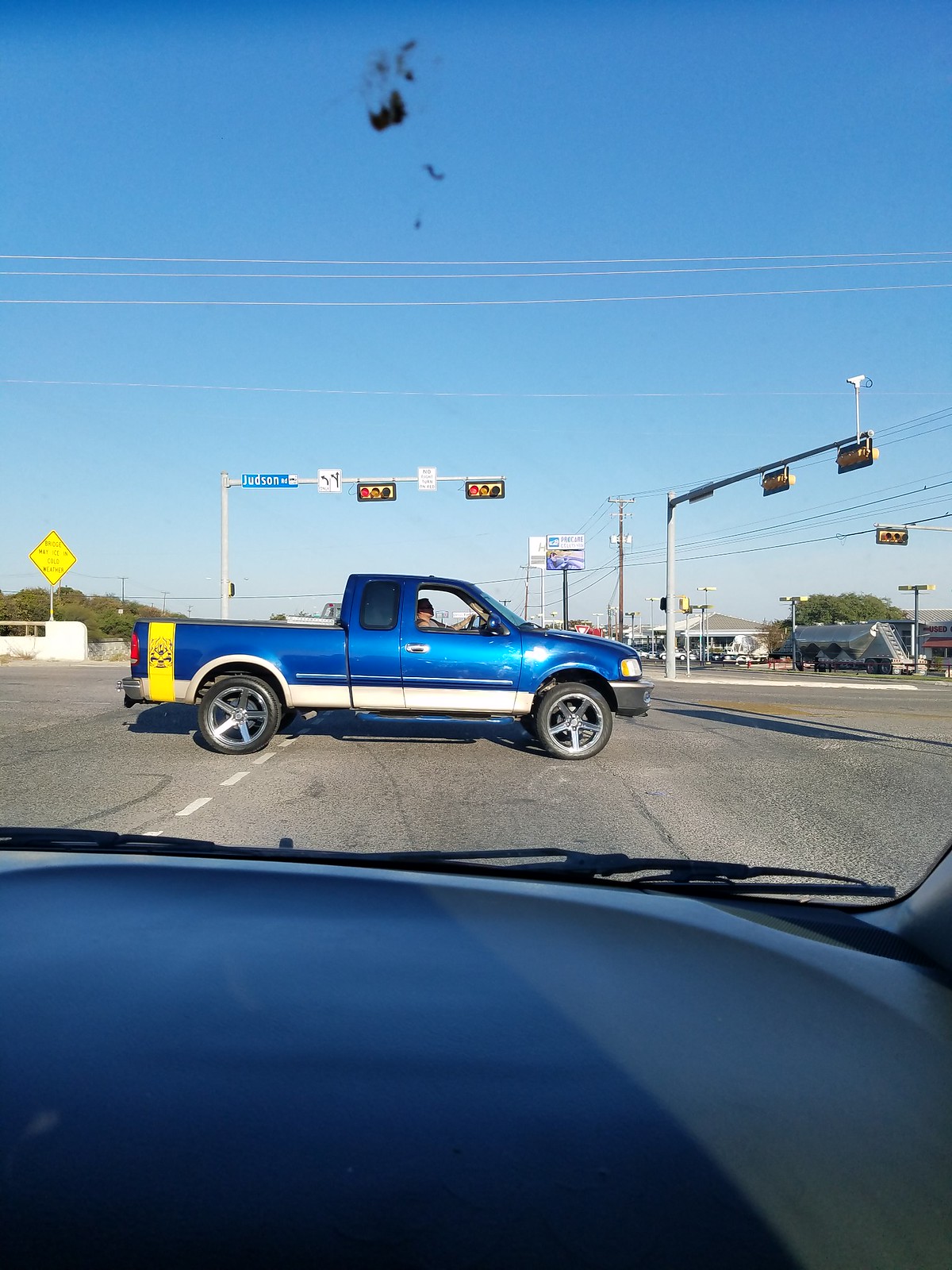The image depicts a scene from inside a car, presumably taken from either the driver's or passenger's seat. The car is stationary at a road junction, and the foreground features part of the dashboard and the start of the side window. Directly ahead, crossing perpendicularly in the middle of the road, is a cobalt blue pickup truck with a yellow line on the back and a white stripe underneath. The truck displays mag wheels and is oriented side-on. Beyond the truck, we can see two traffic signals, both showing red lights; the leftmost lane is designated for left turns, while the neighboring lane offers the option to either turn left or proceed straight. Additionally, the scene includes various streetlights and a blue street sign, which remains unreadable. The sky above transitions from a dark blue at the top to a lighter hue as it reaches downwards, contributing to the overall outdoor setting of this American road intersection.